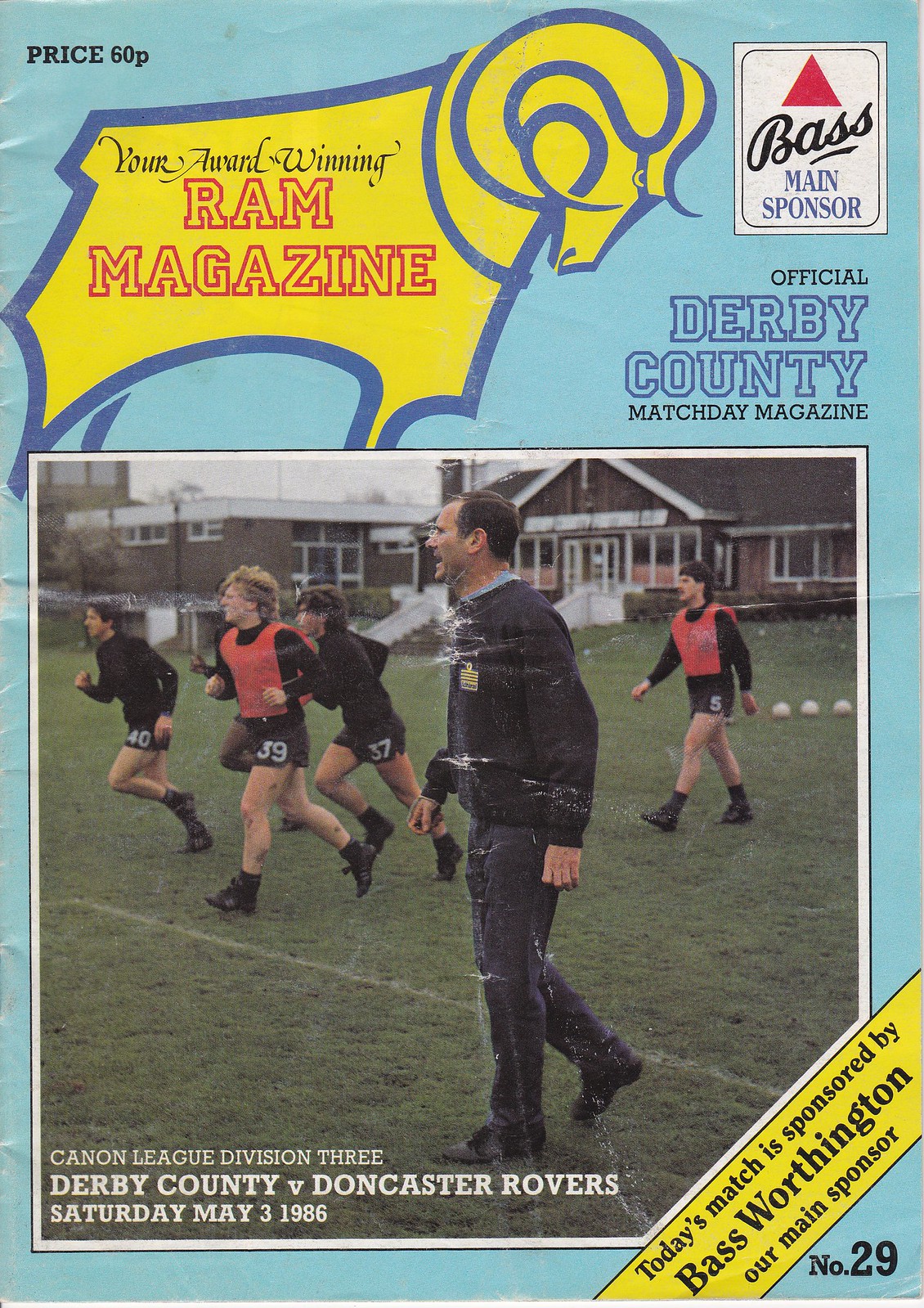This is the cover of "Ram Magazine," the official Derby County Match Day Magazine, priced at 60 pence, sponsored by Bass Worthington. The cover is light blue, with creases and smudges mainly on the left side, top bottom right corner, and middle. A yellow ram, bordered in purple, features prominently at the top, with text reading "Your Award Winning Ram Magazine." To its right, additional text reads "Official Derby County Match Day Magazine."

Below, a central square photograph captures a coach addressing a group of soccer players on a green grass field. The players, some wearing black and white uniforms and others in orange pinnies, are poised attentively. Black shorts with visible numbers such as 40, 39, 37, and 5 signify their preparation. 

At the bottom of the photograph, details of the event are clearly stated: "Canon League Division III Derby County vs Doncaster Rovers Saturday, May 3, 1986." The number "29" is noted in the bottom right corner of the cover, contributing to the detailed and organized layout of this vintage sports magazine cover.